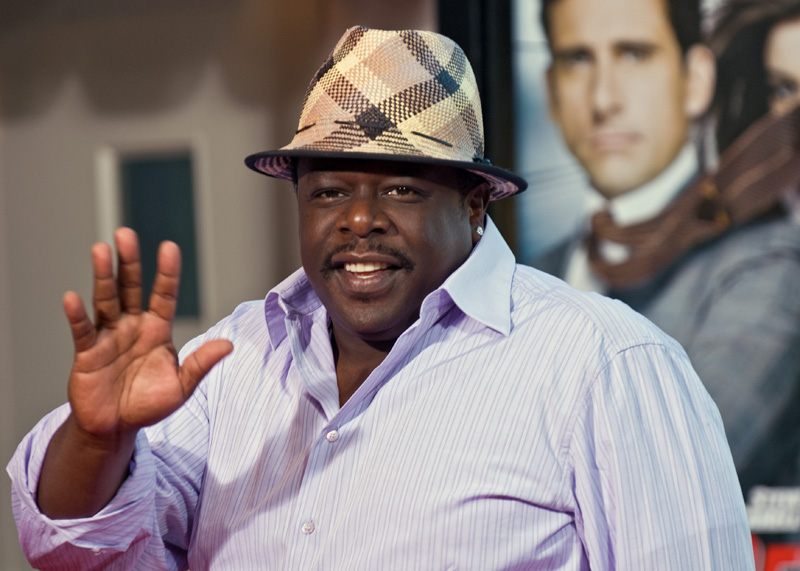The photograph features actor Cedric the Entertainer wearing a button-up, white and blue striped shirt with the top two buttons undone and the sleeves rolled up to mid-forearm. His right hand is extended in a wave, palm facing forward. Cedric sports a black mustache and a round earring, and he tops off his look with a fedora that has a black, white, and tan checkered pattern. The background includes a gray wall on one side and a large movie poster on the right. The poster depicts actor Steve Carell in a gray business coat, white button-up shirt, and a brown tie blowing in the wind. A partially visible woman with dark hair and blue eyes is also on the poster. Additionally, there is a white door with a small window and shadows cast by what might be an awning or overhang.